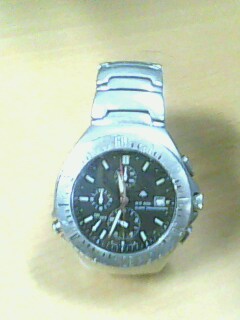A highly detailed photograph showcases an elegant silver metal watch featuring a traditional circular dial. The dial face is adorned with white Roman numerals set against a sleek black background, accompanied by smaller white dashes marking the seconds. On the right side of the dial, there is an integrated calendar displaying both the date and the month. The left side of the watch face houses a smaller circular compass, clearly indicating the cardinal directions: north, south, east, and west. This multifunctional watch seamlessly combines time-telling, navigational, and calendrical capacities, making it both a sophisticated accessory and a practical tool.